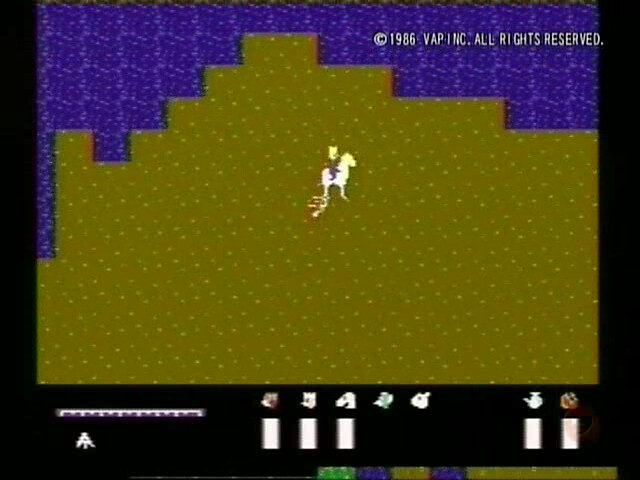This vintage video game screenshot, dated 1986 with a copyright notice from V.A.P., Incorporated, prominently at the top right, showcases classic gaming aesthetics. The central display features a building-shaped outline rendered in olive green with light yellow speckles and subtle light orange shading, providing a textured ground environment. Slightly above the center of the screen, a figure is depicted atop a white horse, poised and facing to the right. At the bottom, a black text section contains several white logos and various status bars. Additionally, a notable gauge with an arrow pointing upward is positioned at the left-hand side of this text bar, subtly indicating gameplay mechanics or character status.